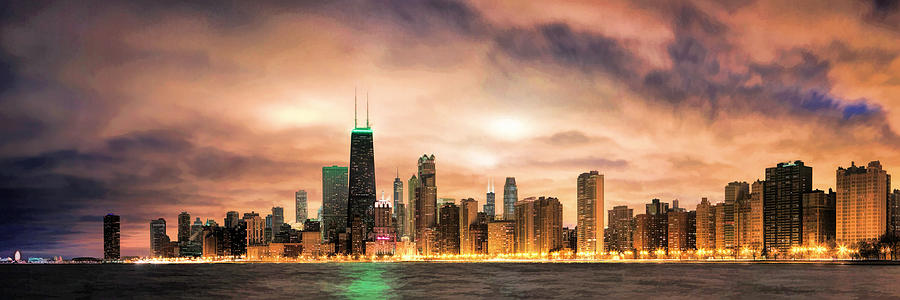This vibrant nighttime photograph captures a sprawling city skyline from across a body of water, possibly depicting New York City or Chicago. The image features an array of skyscrapers of varying heights, the most prominent being a towering structure around 80 stories tall, with two large antennas and a distinctive green light at its top. This green light creates a vivid reflection on the dark water below. The skyline stretches extensively from right to left, illuminated by myriad lights reflecting off a dramatically cloudy sky tinged with orange, yellow, and purple hues. Many buildings glint with a yellowish glow from the city’s streetlights, contributing to the urban nightscape's mesmerizing and reflective ambiance.